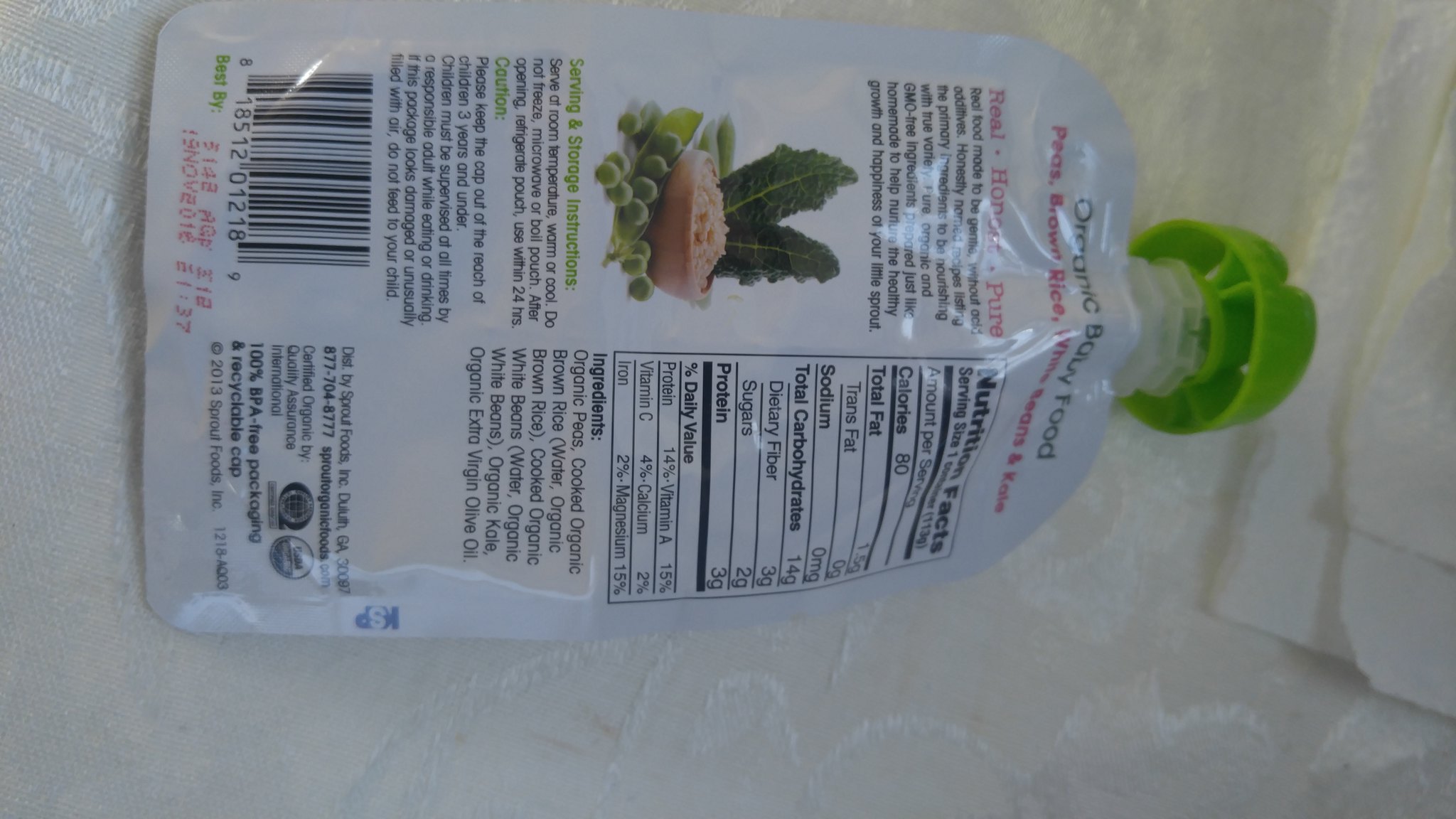This is a color photograph displaying the back of a plastic sachet or bottle resting on a white cloth surface, currently in shadow and appearing grey. A subtle, floral-like pattern is embossed on the cloth. Another piece of cloth is slightly covering the top of the bottle. 

The image is rotated 90 degrees counterclockwise. Upon rotation, a green cap can be seen on the bottle, which features a predominantly white background. A picture of beige-hued food items is present on the left side of the bottle, accompanied by small green round objects resembling peas near the bottom, and large leafy greens at the top, possibly cabbage or lettuce.

Text in black, partially highlighted in red, is situated above and below the picture, though some of it is obscured by glare, making it hard to decipher. A barcode is located at the bottom left, with an indiscernible best before date printed in red beneath it. On the right side of the package, a nutritional chart provides information about the contents. A manufacturer’s logo is placed at the bottom right of the sachet.